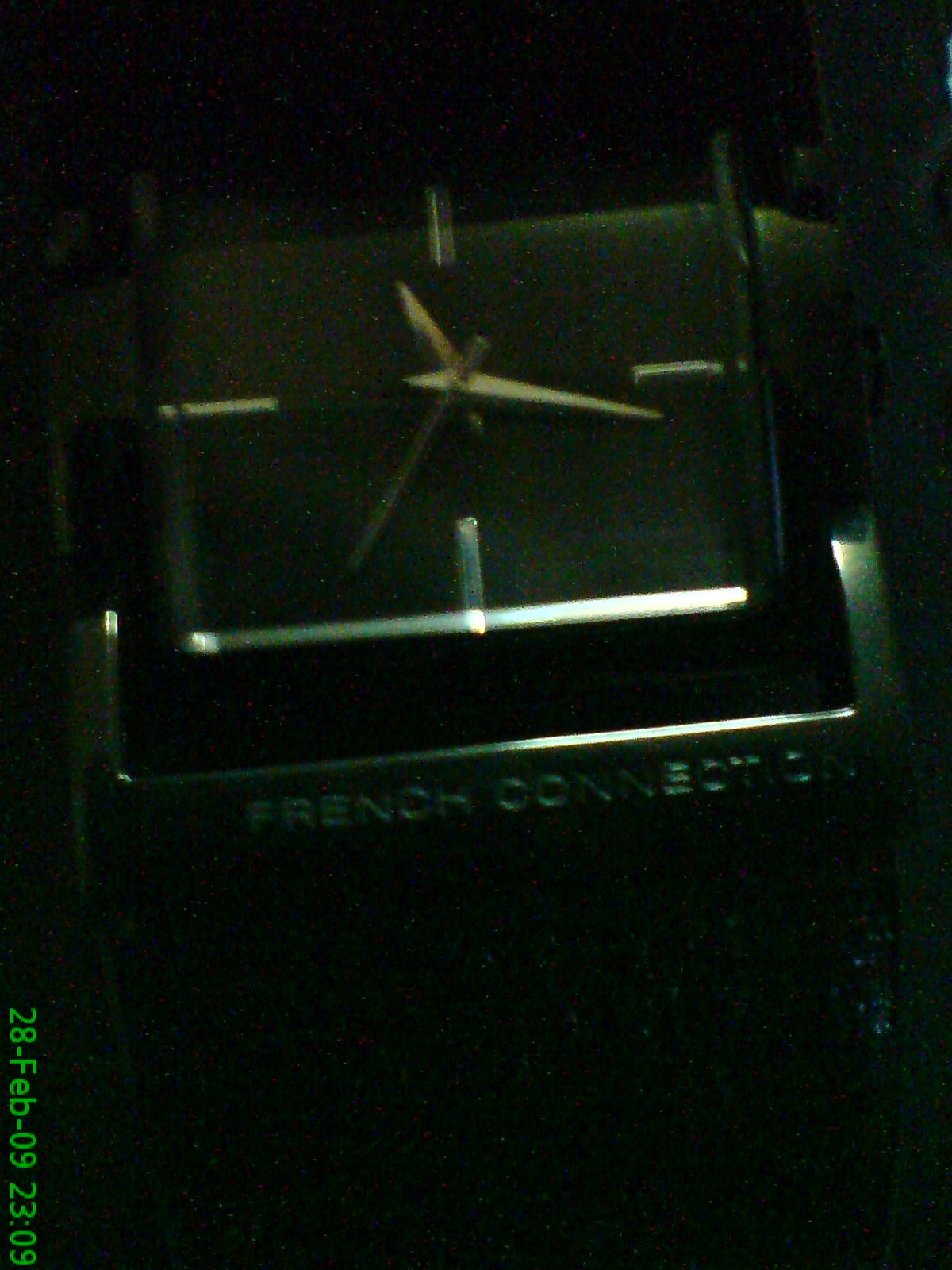This close-up photograph captures the face of a wristwatch, though it is slightly blurry and dark. The watch face is square and minimalist in design. The background is a dark gray, featuring four simple markers at the cardinal positions: one at the top where 12 would be, another to the right at the 3 o'clock position, one at the bottom at 6 o'clock, and one to the left at 9 o'clock. 

The time displayed is approximately 11:17, indicated by two silver-toned hour and minute hands and a longer, silver-toned second hand. The bottom left corner of the watch face bears a light green, vertically arranged inscription: "28-FEB-09 23:09," denoting a date and time. The surrounding area, possibly the band or bezel of the watch, is black, and includes the branding "French Connection."